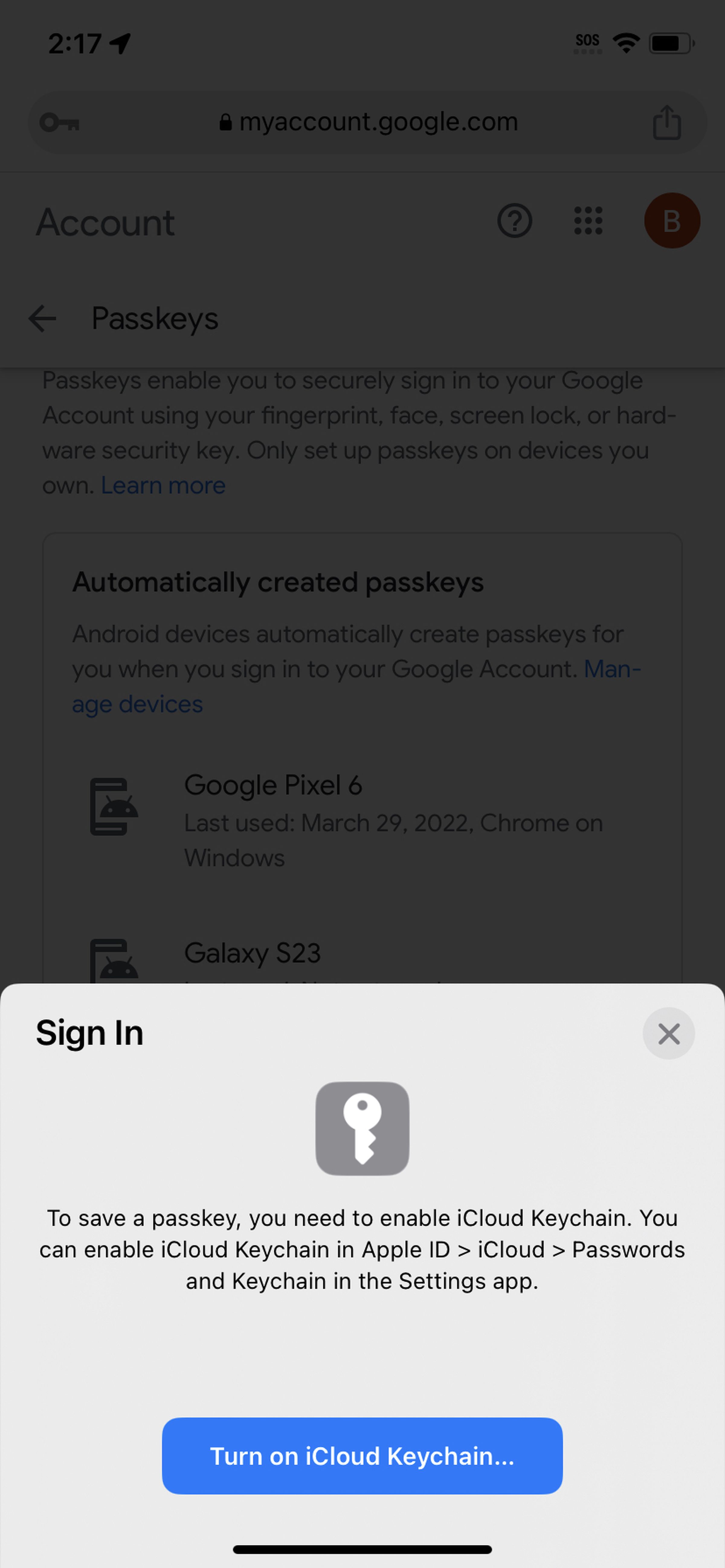This image is a screenshot taken on a smartphone, primarily depicting a sign-in interface related to iCloud Keychain. At the very bottom of the screen, there is a pop-up message that emphasizes the need to enable iCloud Keychain to save a passkey. The message is housed in a gray box featuring a key logo and reads: "To save a passkey, you need to enable iCloud Keychain. You can enable iCloud Keychain in Apple ID > iCloud > Passwords & Keychain in the Settings app." Accompanying this message is a blue button labeled "Turn on iCloud Keychain" and an 'X' button on the right side for closing the pop-up.

In the background, the website displayed appears to be a Google Accounts page, as indicated by the URL "myaccounts.google.com" visible in the address bar at the top. The page is partially obscured but features several elements: the word "Accounts" at the top center, a circular question mark icon, and a grid icon with nine squares. Below the header, there is text regarding passkeys, followed by an option to "Automatically create passkeys," which is described in additional body text. Further down, there is an icon featuring the Android mascot beside a phone illustration, displaying details about the device, such as its name and the date it was last used.